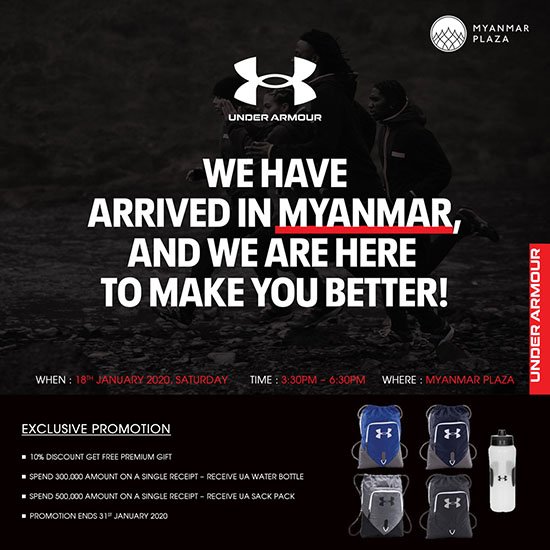This promotional image from Under Armour prominently features a dynamic running scene in the top two-thirds, which is slightly darkened, creating a dramatic effect. The bottom third consists of a solid black background. The main visual depicts a group of runners moving towards the left. At the forefront are two shorter children, their heads visible, followed by a man who is notably taller by about a foot, and behind him, another slightly shorter person.

Overlaying this scene is the iconic Under Armour emblem — the overlapping “U” and “A” — with "UNDER ARMOUR" written in all capitals below it. In the top right corner, a circle encloses a mountain range illustration with the text "MYANMAR PLAZA" in white.

Below the Under Armour logo, in large, bold white capital letters, it reads:

"WE HAVE 
ARRIVED IN MYANMAR,
AND WE ARE HERE 
TO MAKE YOU BETTER!"

This text is accentuated with a red underline.

Running vertically along the right side of the image, white text on a red border states "UNDER ARMOUR". At the lower part of the image, against the black background, small white lettering provides event details, including the date and time in red, with "WHERE" in white adjacent to "MYANMAR PLAZA" also in red. Centered at the bottom, large white text underlined declares "EXCLUSIVE PROMOTION". Below this are detailed offers listed in four squares:

1. Discounts on specific items,
2. Free gifts with purchase,
3. Special limited-time deals,
4. Additional promotional items.

To the right are images of four Under Armour backpacks, arranged two by two, each displaying the Under Armour logo, with an Under Armour water bottle placed to the right of the backpacks.